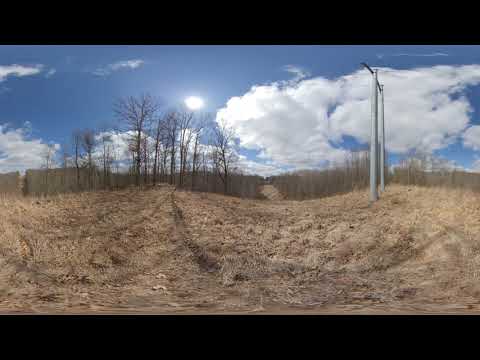In this vivid photographic image set outdoors during daytime, a desolate, arid field stretches across a hilly landscape. The foreground is dominated by barren brown soil and scattered dead grass and bushes, suggesting a late fall or early winter season. On the right side, two green and light gray metal poles stand isolated, unconnected by any wiring. To the left, leafless trees starkly line the edge of the field, accompanied by a densely packed forest in the background whose foliage is indiscernible. The stark, naked trees underscore the season's bleakness. Above, a clear blue sky dotted with puffy white clouds frames a bright, white sun positioned in the middle of the image, enhancing the scene's desolate beauty. The horizon is shaped by gently curving hills, adding to the lifeless and barren atmosphere of the landscape.